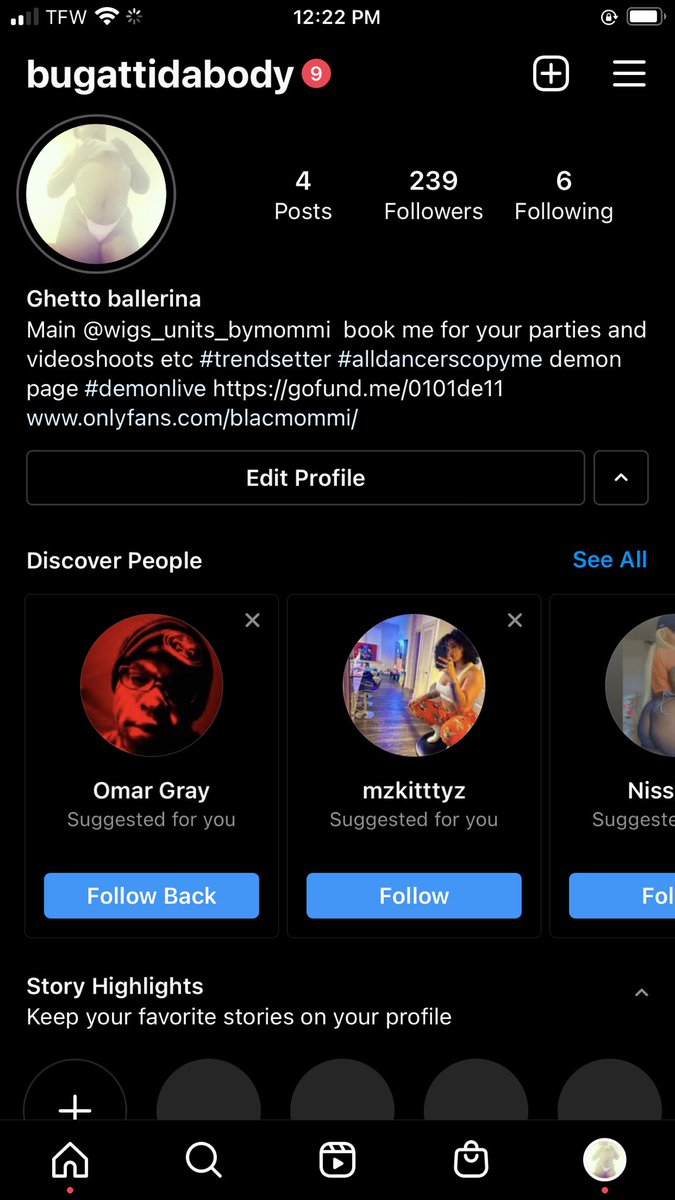**Detailed Caption:**

"At 12:22 p.m., the phone screen displays a partially loaded TFW Wi-Fi signal with two out of four bars and a nearly full battery. The device's carrier is AT&T, and the user appears to be interacting with their Instagram profile. The bio reads, 'Ghetto Ballerina, main at Wigs Unit by Mommy. Book me for your parties and video shoots, etc. Trendsetter—all dancers copy me. Demon page, demon live.' There are direct links to GoFundMe and OnlyFans pages, followed by 'Edit Profile' and 'Discover People' options. Under suggested profiles, 'Omar Gray' and 'Miss Kitty Z' are recommended to follow. The profile highlights story features and has 239 followers and 6 following. The username seems to be 'Black Mommy'."